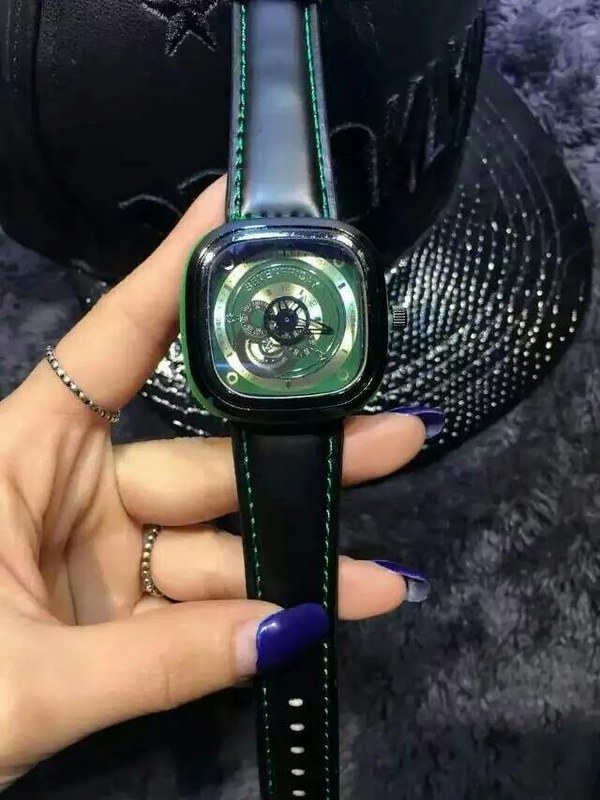A close-up image captures a woman's left hand gracefully holding a digital watch. She has long, manicured nails painted a vibrant blue. The watch, which features a black strap with green stitching along the inseam, is elegantly pinched between her thumb, middle, and ring fingers, with her index finger providing support at the top. The face of the watch is square with rounded edges, showing intricate green gears and a black central gear, giving it a shiny, metallic, and expensive appearance. The background showcases a plush, purplish fabric that adds a touch of luxury to the scene, complemented by a glittering, blinged-out black cap. The woman also wears two stylish rings, adding further elegance to the detailed composition.